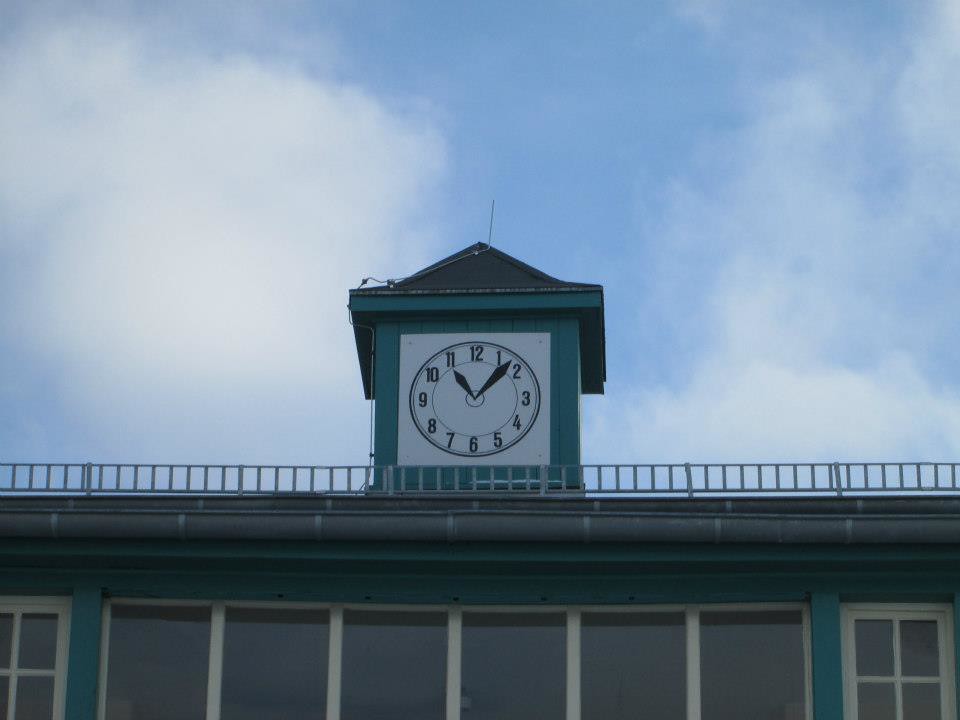This photograph captures a teal-colored building adorned with distinctive white trim around its windows. The trim forms a cross pattern on the outer windows and a vertical stripe on the central ones. Above the windows, a small silver metal railing runs along the top edge of the wall. Surmounting the building is a square room crowned with a gray, triangular roof. Positioned prominently on the front of this room is a classic clock, displaying the time as 11:08. The clock's face features bold black numbers from 1 to 12 set against a white background. The sky above is a soothing blue, accented by a scattering of thin clouds on the right and slightly thicker clouds on the left, adding a touch of dynamism to the serene scene.